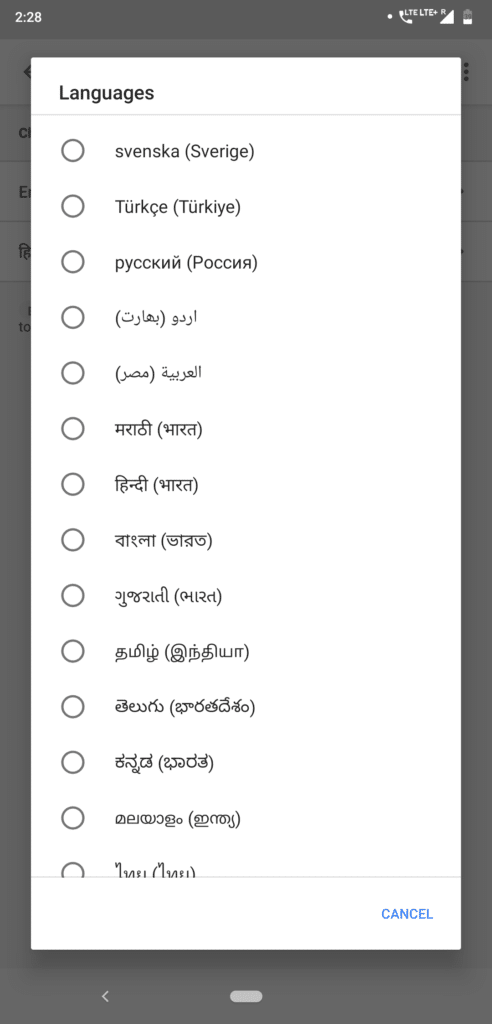The image depicts a mobile application's user interface where a language selection dialogue box is prominently displayed in the center of the screen. The dialogue box occupies most of the view, obscuring the underlying page. The background of the dialogue box is white, and the text is in black. The top three languages listed are in the Latin alphabet, while the rest of the languages appear to be in non-Latin scripts, such as Arabic, Hebrew, or Hindi. There is a rectangular blue "Cancel" button located in the bottom right corner of the dialogue box. The status bar at the top of the screen indicates a strong cellular signal, with the network showing "LTE" and "LTE+". The battery level is around 25%, and the current time displayed is 2:28.